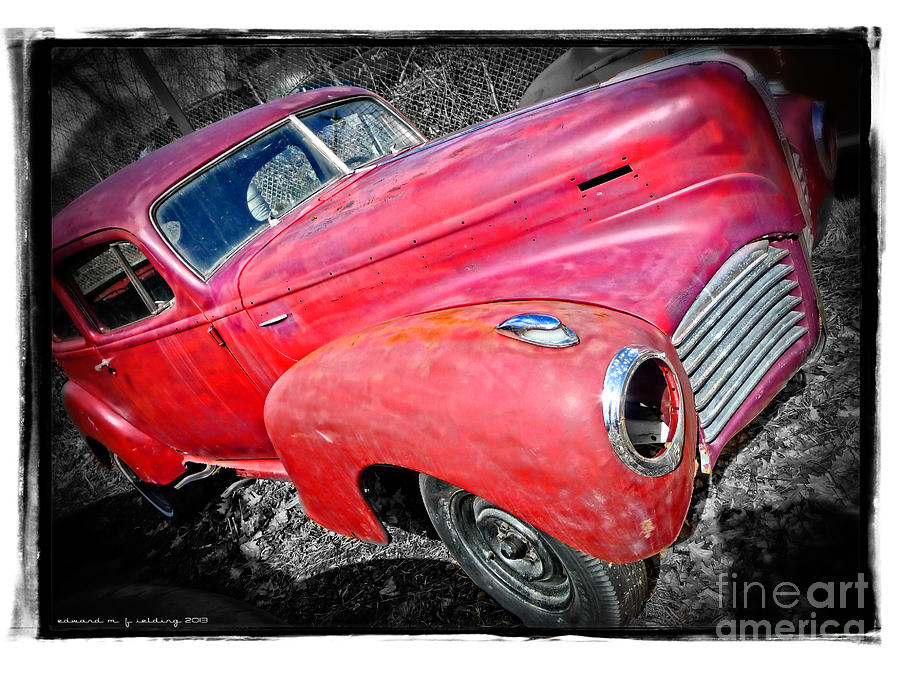The image features an old-timey, classic car with a bulky metal frame and a rusty red, faded paint job that highlights brighter in some areas, particularly the fender and hood. The vehicle is missing its headlights and one of the side windows, but it still has its windshield and a silver grille. The charcoal-colored tires contrast sharply against the ashen or coal-like ground, creating a black-and-white effect that makes the car’s rusted red color stand out more vividly. A silver handle is visible on the passenger door, contributing to the nostalgic feel of the car. In the background, a chain-link fence is discernible, adding to the image’s rustic atmosphere. The bottom right corner of the image is marked with "Fine Art America." The photograph appears to be edited to enhance the faded and distressed look of the car, with the monochromatic ground and fence serving as a stark contrast to the vibrant, albeit weathered, color of the automobile.